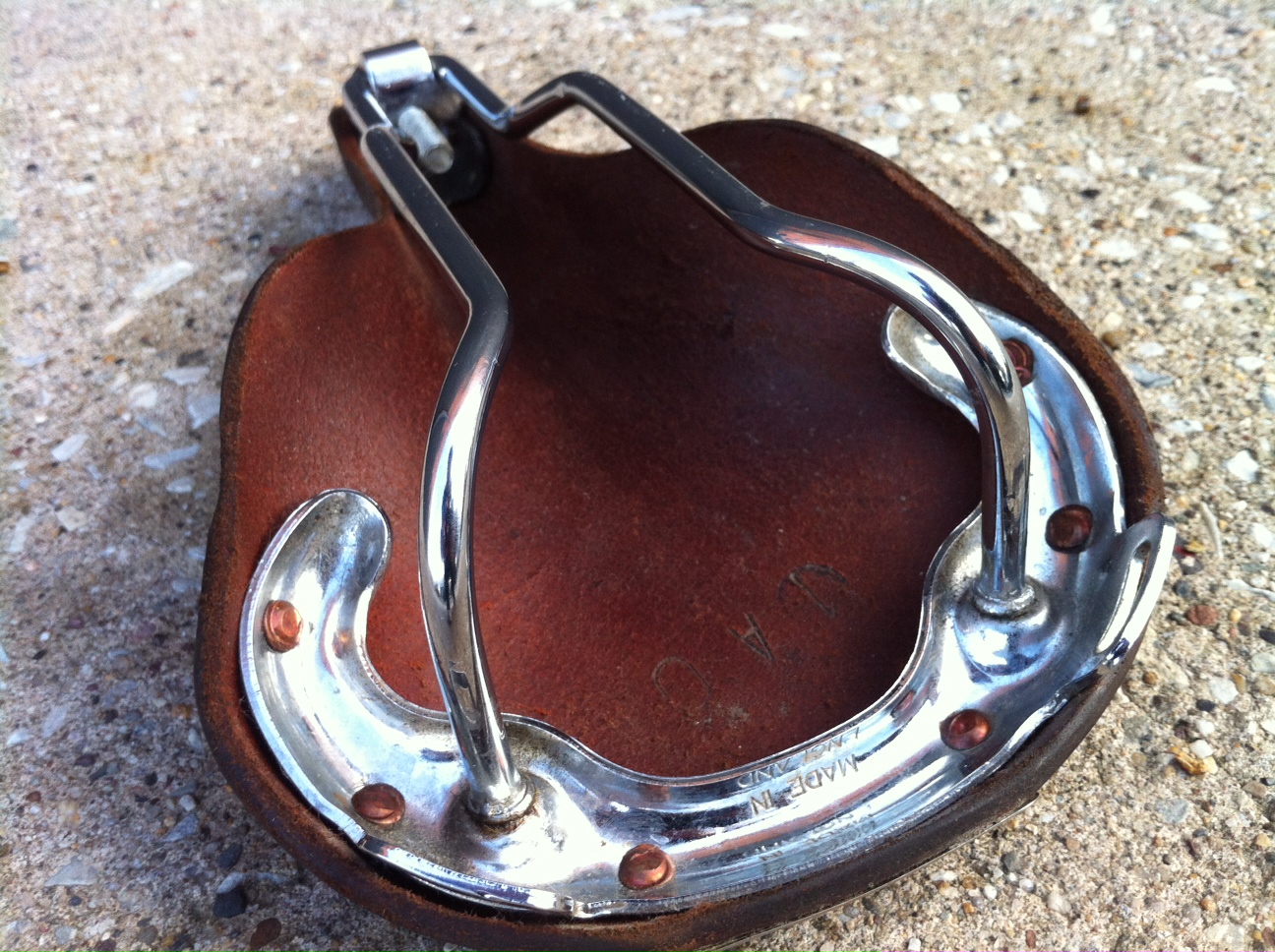This is an image of the underside of a bicycle seat, which has been removed from the bike and placed on a gravelly or stone-covered ground. The seat is made of brownish-reddish leather with a metallic base. The metallic components include a stainless steel or cast metal structure, with six copper bolts securing the leather to the frame. The image reveals text imprinted on the metal that reads "Made in Mexico." The ground underneath the seat has a mix of white, orange, and brown stones scattered across it, giving the impression of a rough pavement or driveway.